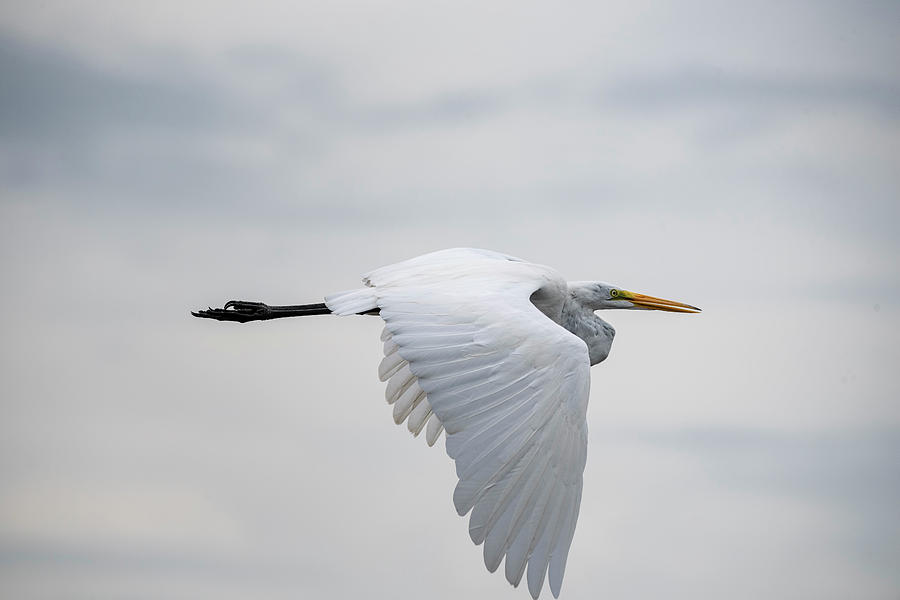This is a highly detailed photograph of a white stork in mid-flight against a backdrop of cloudy, white-grayish sky. The bird is pictured flying from left to right, showcasing its impressively long wingspan and sleek form. The stork's wings are white, and the photograph captures the intricate details of its ruffled feathers, which create a loopy pattern at the edges. The beak is long, sharp, and yellow with red highlights, and its eyes are vividly defined, adding to the overall sharpness of the image. The bird has black legs and feet, which are outstretched behind it as it soars gracefully through the sky. The cloudy background contrasts beautifully with the clear and vivid depiction of the bird, making this an exceptionally excellent photograph.